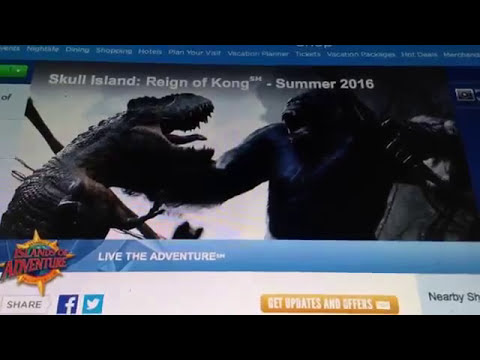The image, likely a screenshot from a theme park's website, prominently features an intense battle between King Kong and a gray T-Rex, both roaring with wide-open mouths, amidst a backdrop suggestive of Skull Island. The headline "Skull Island, Reign of Kong, Summer 2016" stretches across the top, hinting at a new attraction. Above the main image, links like Dining, Shopping, Hotels, and Plan Your Visit are displayed against a blue background. Below, a banner advertises "Islands of Adventure" with the tagline "Live the Adventure." The lower section of the image includes share icons for Facebook and Twitter, and a clickable orange button labeled "Get Updates and Offers."